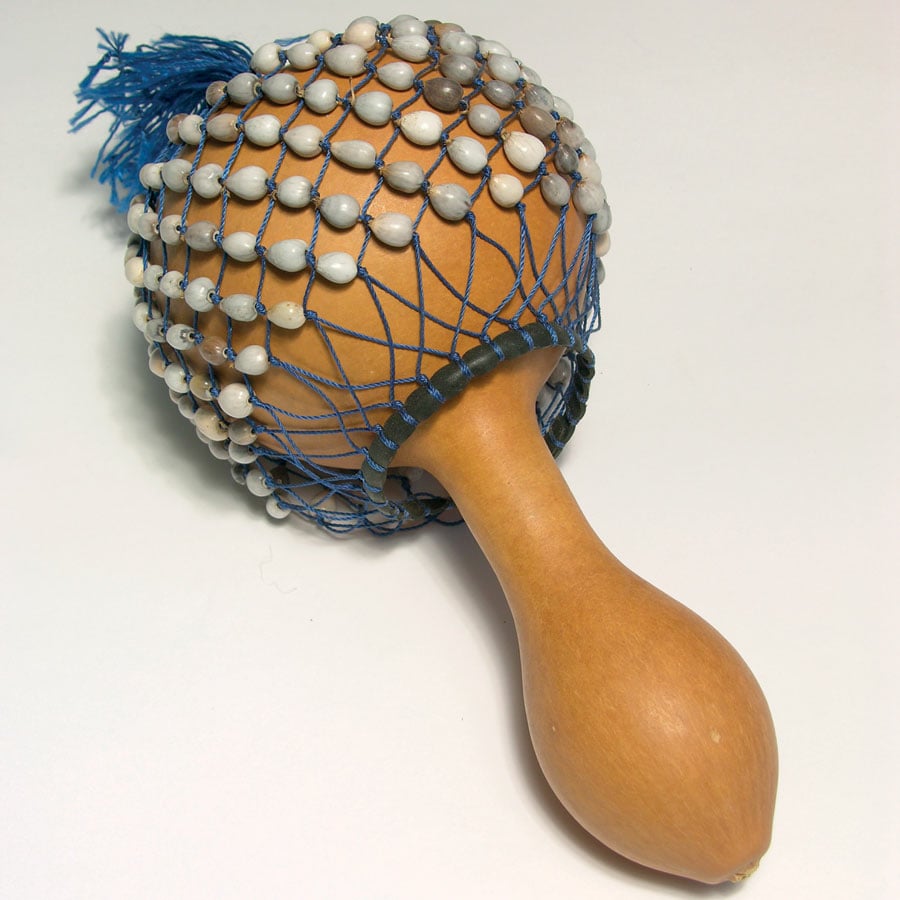The image features a musical instrument prominently displayed on a white background in a vertical, rectangular frame. Positioned diagonally from the top left to the bottom right, the instrument begins with a large, spherical wooden gourd, approximately the size of a large baseball, tapering into a cylindrical handle that broadens slightly towards the end. The gourd is enveloped in blue netting adorned with white beads arranged in diagonal rows. At the top of the netting, blue fringe or tassels accent the design, while dark gray beads cinch the netting tightly around the bottom of the gourd. This percussion instrument, reminiscent of a maraca, is designed to be shaken, creating rhythmic sounds often utilized in Latin and Caribbean music to keep time.